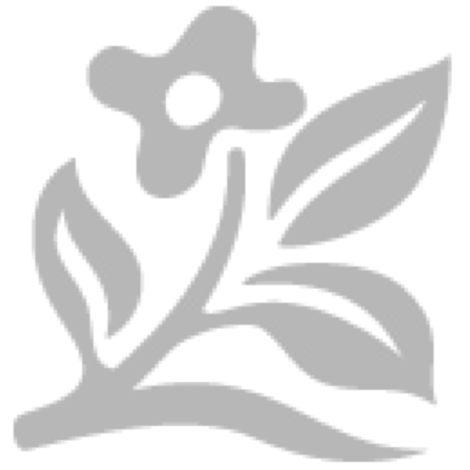A highly detailed nature photograph captured outdoors during the day showcases a close-up view of a fruit tree. The image, vertically rectangular and taken in full color under natural light, brings into focus a single, intriguing fruit hanging from a white-brown branch. The fruit, roughly circular in shape, has a dull yellow color and is speckled with white dots. It appears to be split open, revealing a whitish interior. The tree's leaves, displayed prominently around the fruit, exhibit a variety of colors and textures. Some leaves are a vibrant green, while others transition to yellow-green and then to a reddish-brown hue. The leaves themselves are oval with serrated edges and are longer than they are wide. The tops of the leaves are green, whereas the undersides are red, adding to the intricate detail of the image. The surrounding background is slightly blurred, hinting at more foliage of the same kind, but no additional fruits are visible. This rich interplay of colors and textures makes the photograph a captivating study of nature’s details.